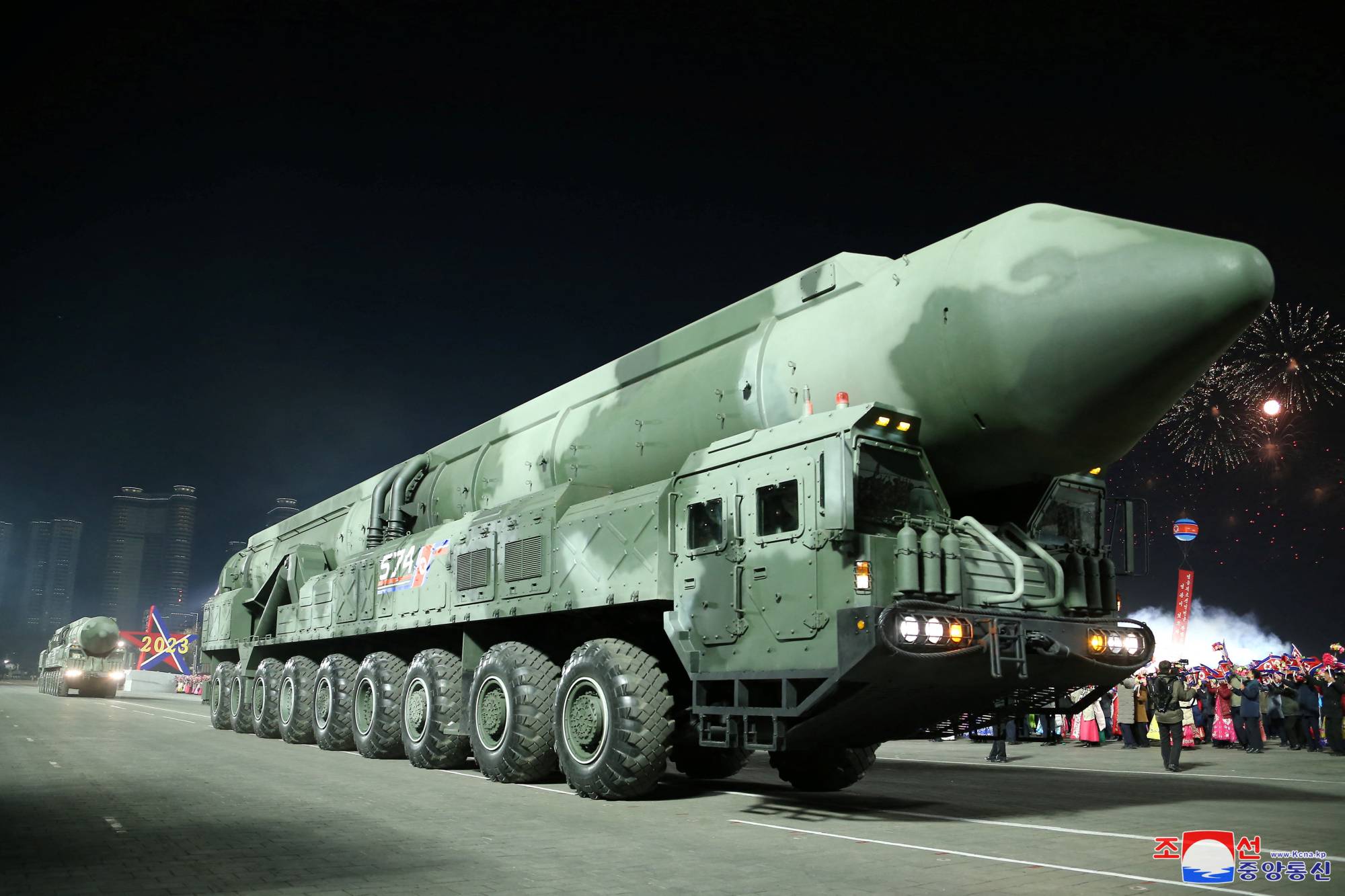The image depicts a massive camouflaged military vehicle, likely part of a North Korean military parade, traveling down a road at night. The vehicle is long, resembling a hybrid between a truck and a tank, equipped with an intercontinental ballistic missile (ICBM) on top. It has at least ten wheels on each side, making its substantial size evident. The dark green and light mint green camouflage blends with the nighttime setting, where fireworks illuminate the sky. Another similar vehicle follows closely behind. In the background, several people can be seen, likely witnessing the parade or demonstration, with soldiers maintaining order. Banners with Korean text and a star-shaped banner with "2023" in yellow lettering are visible, along with a red, white, and blue logo featuring foreign lettering in the bottom right corner. The overall scene strongly suggests a New Year's celebration marked by a military display in North Korea.